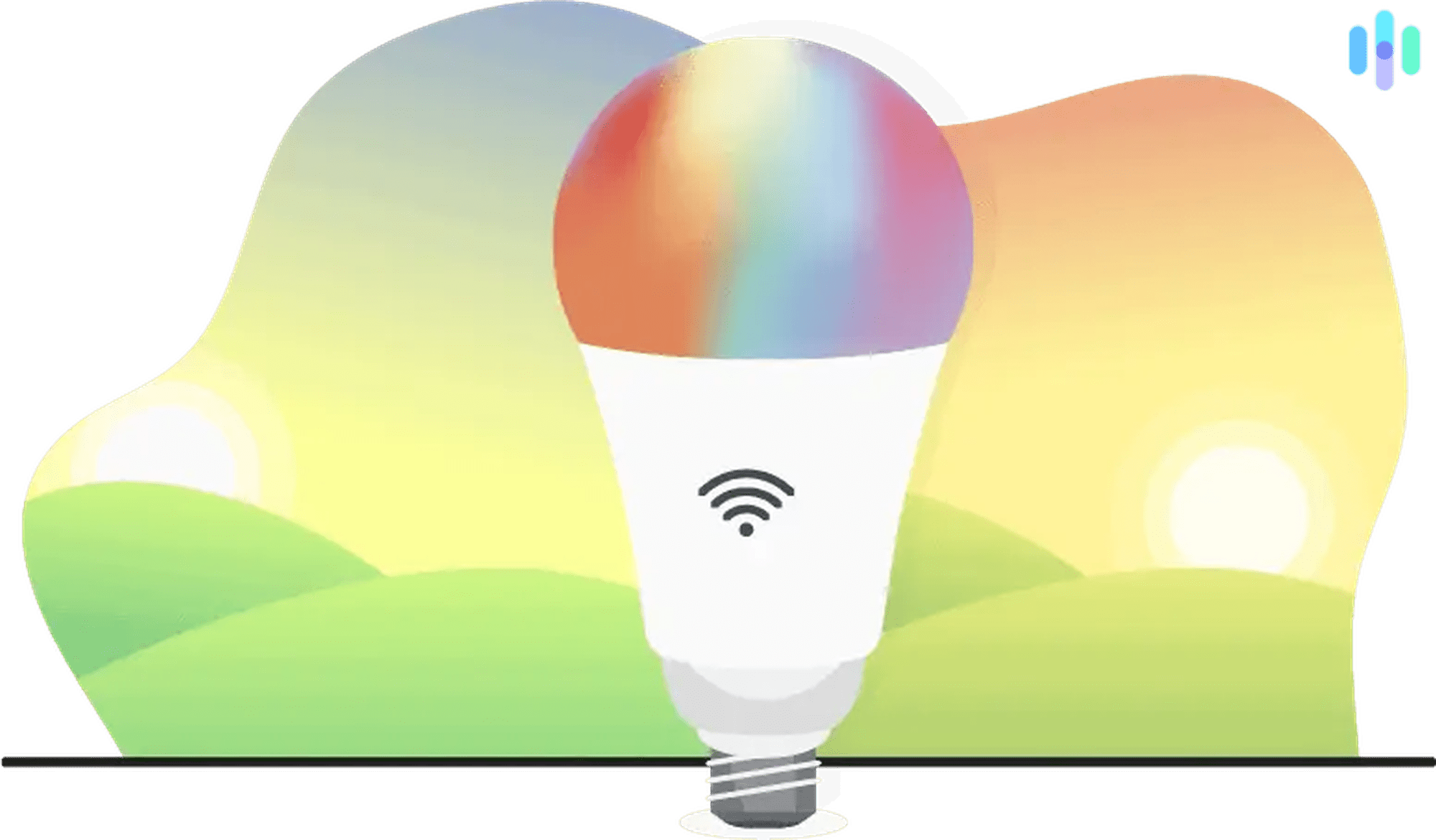The image features a detailed drawing of a light bulb with a multicolored glow where the light would emanate. The bulb's luminous portion displays a spectrum of colors, including orange, red, golden yellow, turquoise, green, violet, and purple. The middle section of the bulb is white with a Wi-Fi symbol drawn on it, while the base that screws in is gray with white diagonal stripes. The bulb is set against a backdrop that appears digitally rendered, showing a vibrant landscape composed of green hills and a sky filled with rainbow-like hues. The sky also features two shining suns, one on the left and one on the right. Additionally, there are blue and peach-colored humps and several white semi-circles, with three elongated ovals in varying shades of blue and gray positioned in the upper right corner of the image.